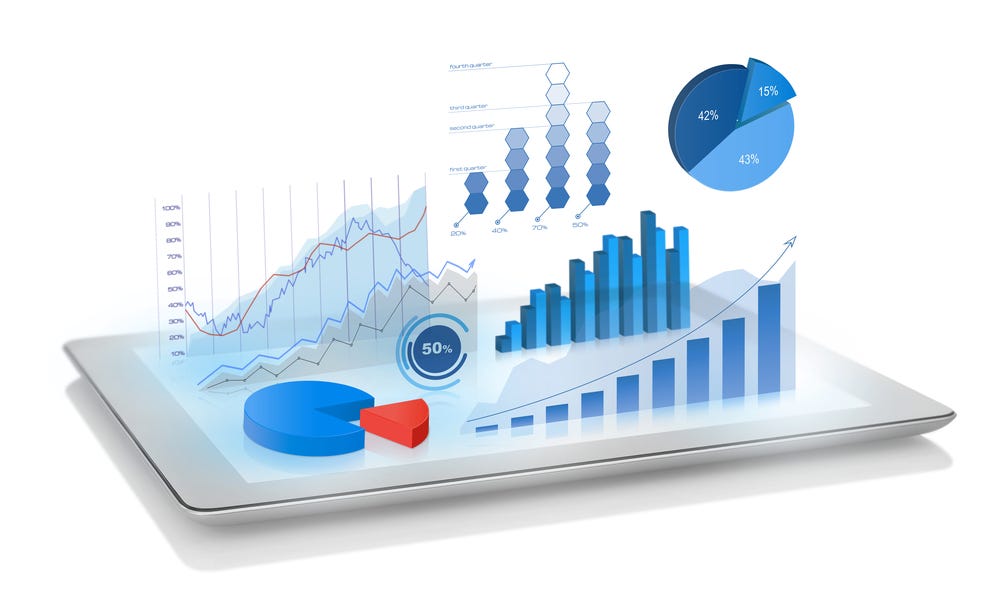This is a diagonal, horizontal rectangular image of a three-dimensional graphic representation, projected upward from an iPad base with no outer border. In the front left corner, there is a partially circular blue raised area with a pie-shaped cutout filled by a red switch. This section is part of a blue pie chart with an orange wedge labeled 50 percent. Adjacent to this is another 3D graph with axes and labels depicting three lines that rise and fall. Behind these elements, there is a complex array of vertical lines and an overarching arrow, leading to more vertically oriented bar graphs in dark and light blue shades. Additionally, another pie chart in this section depicts divisions of 42 percent dark brown, 43 percent light blue, and 15 percent medium blue. The entire scene includes various types of charts such as line graphs, pie charts, and a hexagon-patterned graph, predominantly in shades of blue with occasional red elements.